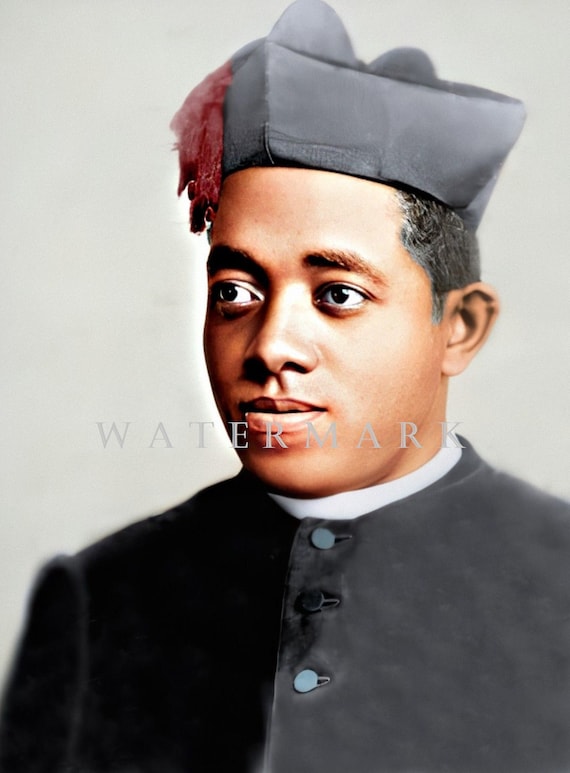This image, which may be a photorealistic painting or a stock photo, features a headshot of a black man, possibly with historical or religious significance. He is dressed in a detailed outfit reminiscent of a high-ranking official or a member of some religious sect. He wears a distinctive black, brimless cap with a red band or tassel on the left side, which evokes a Napoleon-style hat. His expression is serious and he gazes to the left, his lips firmly closed. His short black hair is visible under the cap.

The man is attired in a black, high-buttoned jacket with three buttons, over what appears to be a white shirt or possibly a priest collar. The buttons on the jacket are mentioned to be either silver or blue. The background of the image is gray, and a gray watermark text, reading "WATERMARK," is prominently displayed across the image, just below the man's lips. The composition is detailed down to his chest area, focusing on his somber expression and meticulously described attire.